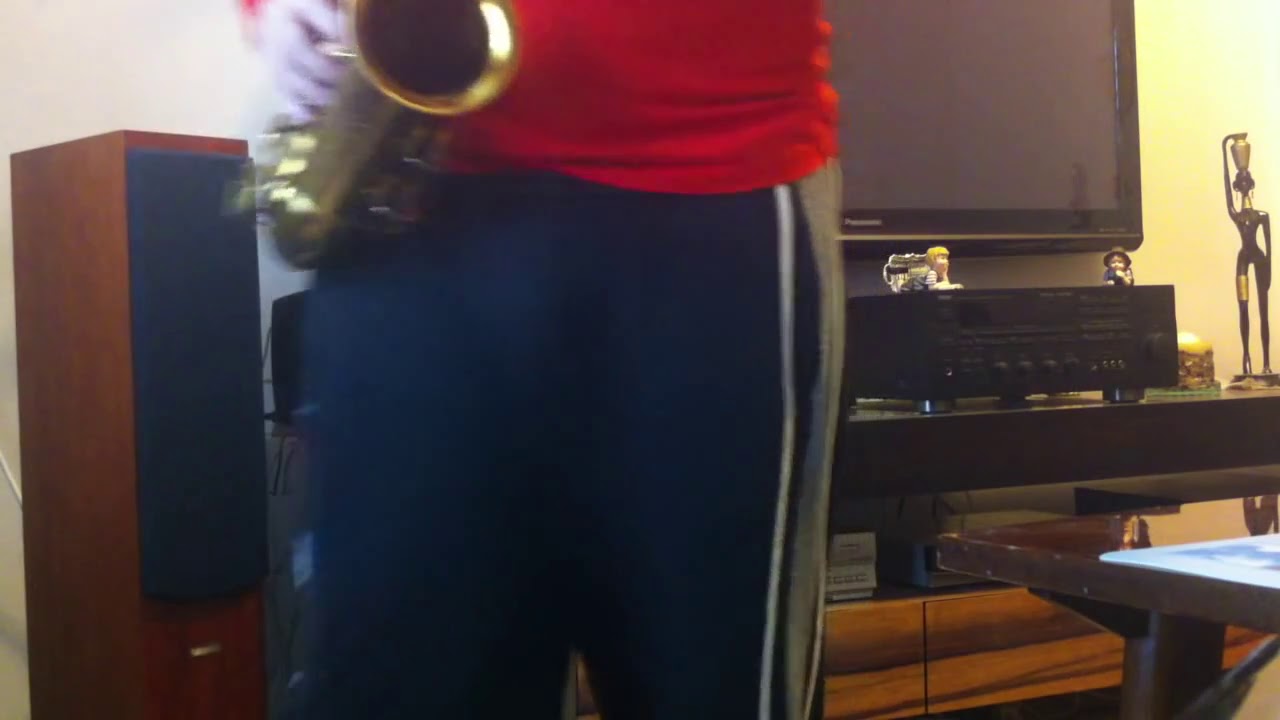A blurry photo captures a man from the waist down wearing blue sweatpants with a white and gray stripe, and a red shirt, up to his midriff, while he holds and possibly plays a saxophone. His fingers are positioned on the saxophone keys, suggesting he might be practicing. The scene is set in a living room adorned with various eclectic items that suggest a shared living space. Behind him, against a yellowish wall, there's an old-school television atop a stereo system and several wooden and black-faced speakers, some of which are quite large, reaching about three feet in height. A wooden shelf beneath the TV holds multiple DVR players and speaker units. The room also includes an African statue of a woman, and several small statues resembling Precious Moments figurines. To the man's left is a rusty coffee table, while to his right, additional speaker cabinets and possibly a tuner speaker or stereo system are arranged. This cluttered yet character-filled background highlights a mixture of personal and possibly shared decor.